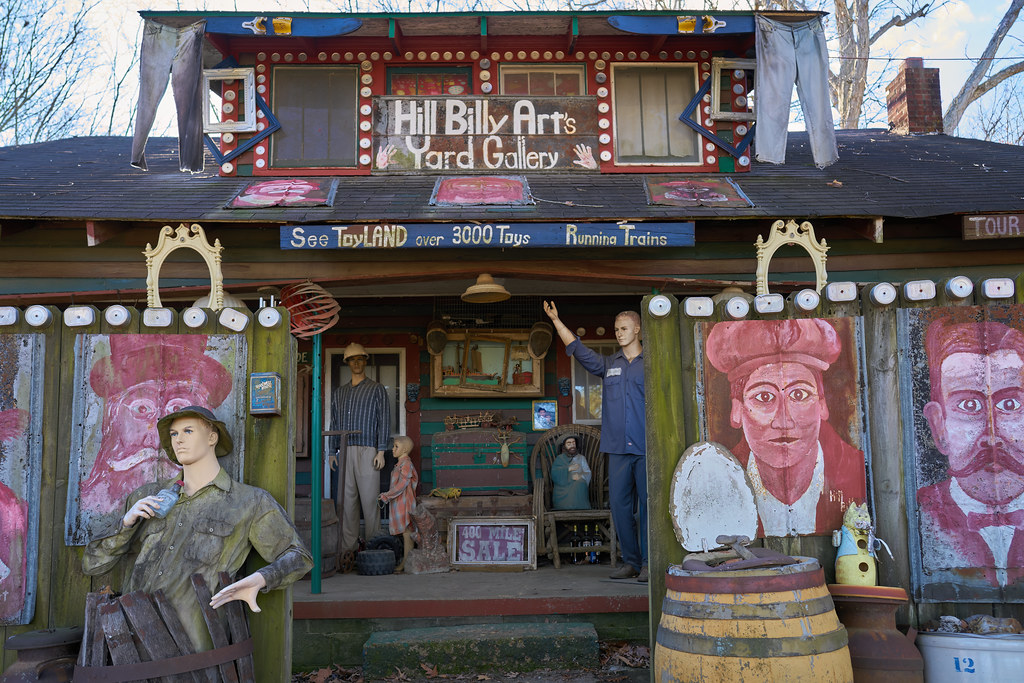This landscape-oriented color photograph captures the eclectic and vibrant exterior of a two-story folk art gallery known as "Hillbilly Arts Yard Gallery." The building, resembling a quaint old house or hut, is adorned with a myriad of unique decorations and artwork. Prominent signs on the second floor read "Hillbilly Arts Yard Gallery" and "See Toyland Over 3,000 Toys Running Trains." Blue jeans hang from either side of the gable roof, adding to the quirky charm.

The ground floor features a porch entry flanked by various characters and knickknacks. On the left, we see a wall adorned with hand-drawn paintings, including close-ups of people such as a man in a suit with a bowtie and mustache, and an old prospector. Sitting in front of this wall, a mannequin dressed in a military uniform sits in a barrel, sipping from a whiskey bottle. To the right of the entrance, more mannequins are posed, including one in all blue with arms extended skyward. 

Adding to the whimsical atmosphere, various objects like a ceramic cat, a vibrant drum with a yellow body and red-green stripes, a dustbin marked with the number 12, and an open commode lid are scattered around. The porch itself is populated with antique-clad mannequins, including a small child figure and an elderly figure, as well as other items like photo frames, paintings, and lights, creating an overwhelming yet intriguing visual feast. The sky and barren trees in the background emphasize the outdoor setting of this peculiar and captivating gallery.